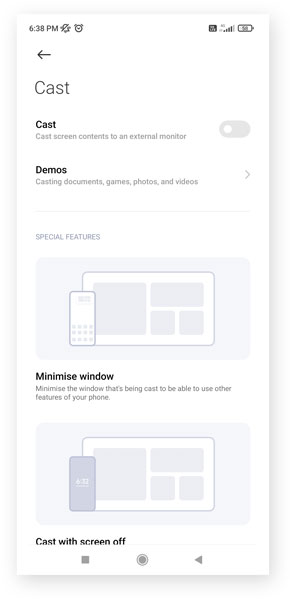This screenshot from a cell phone features a white background in the top left corner, displaying the time as 6:38 PM. At the very top, cell phone signal strength and a battery indicator are visible. 

To the right of the time, there is a bell icon with a diagonal line through it, symbolizing the silent mode, and an alarm clock icon. Below these indicators, a left-pointing arrow appears on the far left, next to the word "Cast." 

The following text reads: "Cast screen contents to an external monitor," with a gray on and off toggle switch to the right, which appears to be turned off. 

Underneath, there is a heading labeled "Demos," followed by a description that says: "Casting documents, games, photos, and videos." A right-facing arrow is present at the far right side here. 

Further down, the label "Special features" appears, with light blue illustrated boxes depicting a cell phone and its screen. The first box includes text stating: "Minimize window - Minimize the window that's being cast to be able to use other features of your phone." 

The bottom box shows another drawing of the phone and screen with the accompanying text: "Cast with screen off."